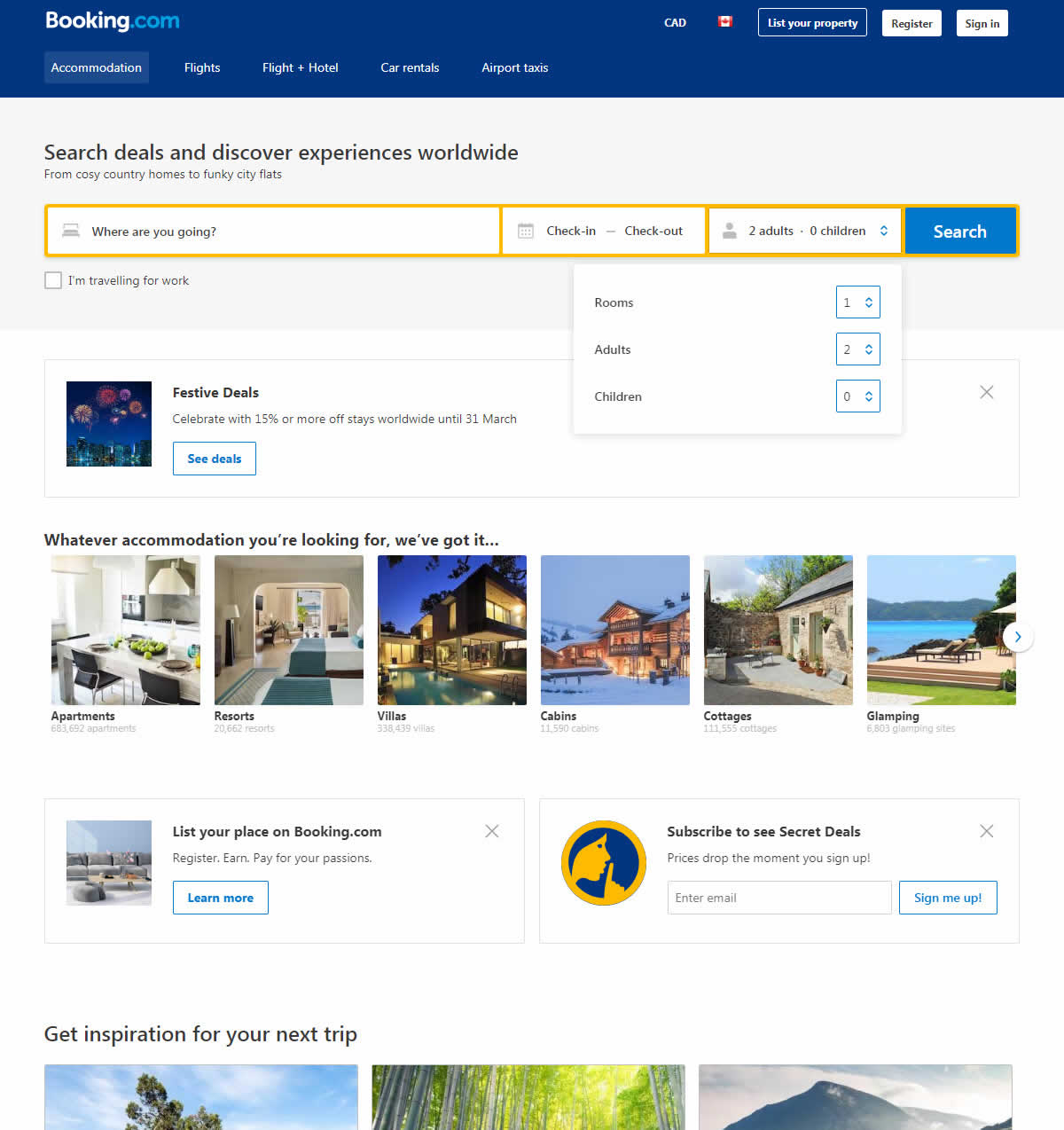The image displays a Booking.com webpage with a distinct blue border at the top. On the left side of this border, the company's logo is prominently featured, consisting of "booking" written in white font and "dot com" in turquoise blue font. In the upper right-hand corner, there are two clickable white boxes: one labeled "Register" and the other "Sign Up." The background of this section is a very light gray, providing a clean and calming aesthetic.

The top headline of the webpage reads, "Search deals and discover experiences worldwide." Below this headline, there is a search box where users can enter their travel details, including the destination, check-in and check-out dates, the number of rooms, and the number of adults and children. A blue "Search" button is positioned prominently to initiate the search.

Directly beneath the search box, there are two rows of photographs showcasing various travel locales. The top row includes images of the interiors of rooms, an exterior view, and a scenic photograph featuring a lake and mountains. Below this row, three partially visible photos can be seen, hinting at a mountain, a forest, and a blue sky with the top of a tree peeking in. The lower portion of these images is cut off, making it difficult to discern the full content.